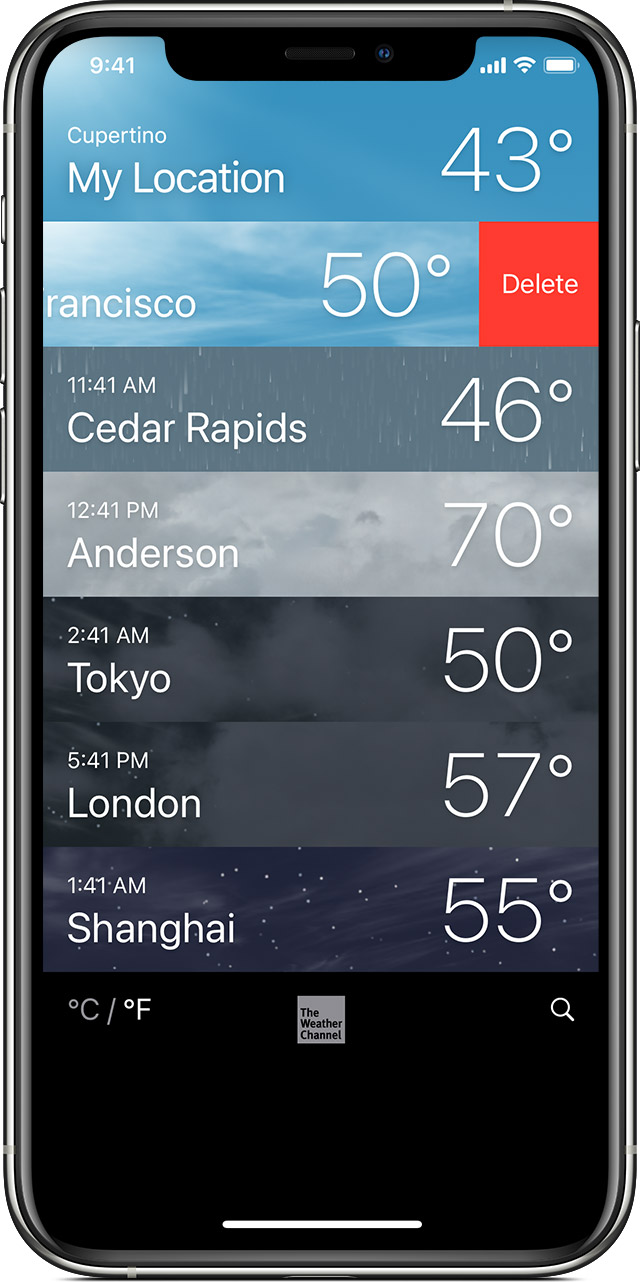The image appears to be a screenshot of a smartphone display, showing a detailed weather and time widget layout. The device is oriented vertically.

At the very top left-hand corner, the time reads 9:41 in white text. The top right-hand corner displays full cellular reception with five bars, a full battery icon, and active Wi-Fi.

The main content is divided into seven sections:

1. **Cupertino**: The background is light blue. On the left side, in smaller white text, it reads "Cupertino," and in larger white font next to it, "My Location." Beside this, the temperature is listed as 43°F.

2. **San Francisco**: Below Cupertino, there's a smaller section with a partly cloudy sky background. It shows "San Francisco" on the left and "50°F" on the right. Next to the 50°F, there's a red box with "Delete" in white text inside it.

3. **Cedar Rapids**: The background resembles a rainy scene. Time shows as "11:41," and on the left, "Cedar Rapids" is written with the temperature listed as 46°F.

4. **Anderson**: Featuring puffy gray clouds, this section reads "12:41" on the left, "Anderson," and a temperature of 70°F.

5. **Tokyo**: Displaying a starry night sky with some gray clouds, this part shows the time "2:41 a.m.," with "Tokyo" listed and a temperature of 50°F.

6. **London**: This section has a similar background to the previous Tokyo section. The time is "5:41 p.m.," with "London" and a temperature of 57°F.

7. **Shanghai**: With a clear purplish-blue night sky, this section displays the time "1:41 a.m.," "Shanghai," and a temperature of 55°F.

All the sections together suggest the diverse weather conditions and times in various cities around the world, likely indicating winter based on the temperature readings.